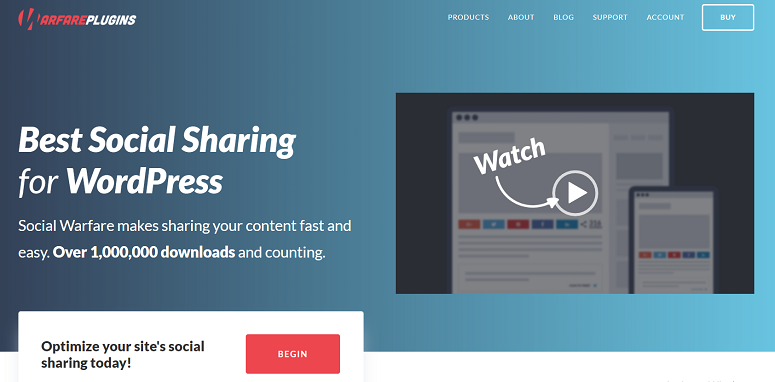The background of this image features a gradient that transitions from light blue on the right side to slightly darker blue on the left side. In the top left corner, the text "Warfare Plugins" is prominently displayed, with "Warfare" written in orange and "Plugins" in white. All other text on the image is also in white.

In the top right corner, there are navigation tabs labeled "Products," "About," "Blog," "Support," and "Account." Additionally, there is a "Bypass" button at the top right.

Centered to the left side of the image, a headline reads "Best Social Sharing for WordPress." Below this, a subheadline states, "Social Warfare makes sharing your content fast and easy," followed by a bolded statistic: "Over 1 million downloads and counting."

At the bottom left, black text urges the viewer to "Optimize your site's social sharing today." Below this message, a red button with white text invites users to "Begin."

To the right of the central text section, there is an embedded video element. Above the video, the word "Watch" is written with an arrow pointing towards a white play button. The video thumbnail displays an interface on both a tablet and a smartphone, providing a visual representation of the product's functionality.